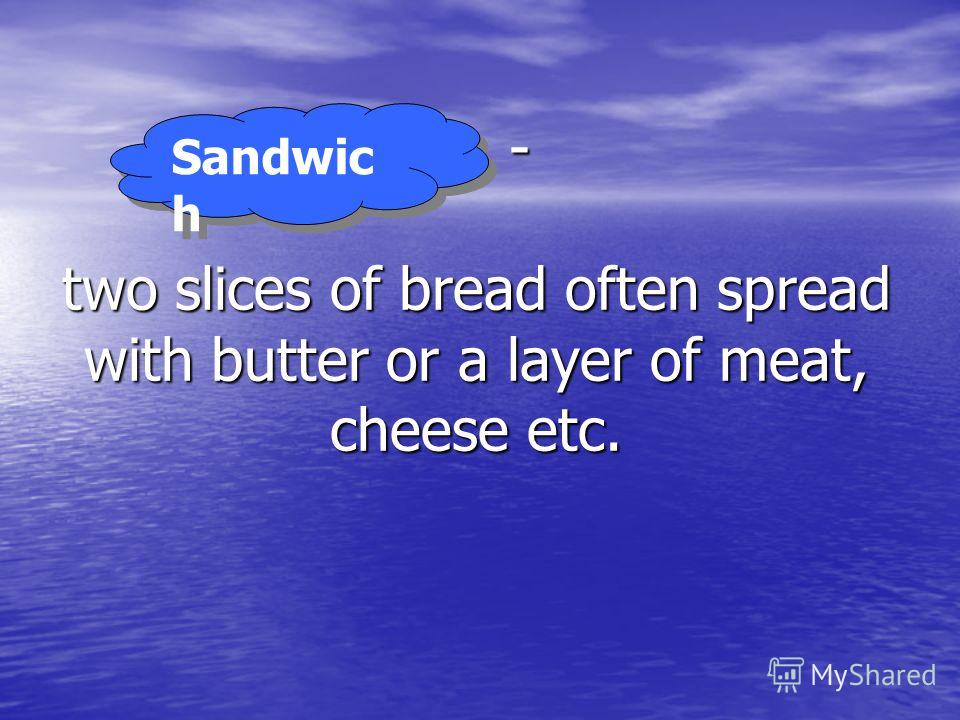The image resembles a presentation slide with a computer-generated, scenic background featuring a vast, calm body of ocean water at the bottom, subtly rippling from the wind, and a serene, partly cloudy sky above. The sky, tinted in shades of blue, is scattered with thin, wispy white clouds, while the water reflects some of this white hue. Dominating the center of the image, there's a focal point of text. In the upper left corner, an illustrated, bright blue thought bubble outlined in black contains the word "sandwich," although the letter "H" is slightly outside the bubble, suggesting a lettering limit. Just below, the definition reads: "two slices of bread often spread with butter or a layer of meat, cheese, etc." The image also includes the words "my shared" in white in the bottom right corner, paired with a small logo of an easel. The predominant colors in the image are purple, various shades of blue, white, and subtle touches of yellow and gray.